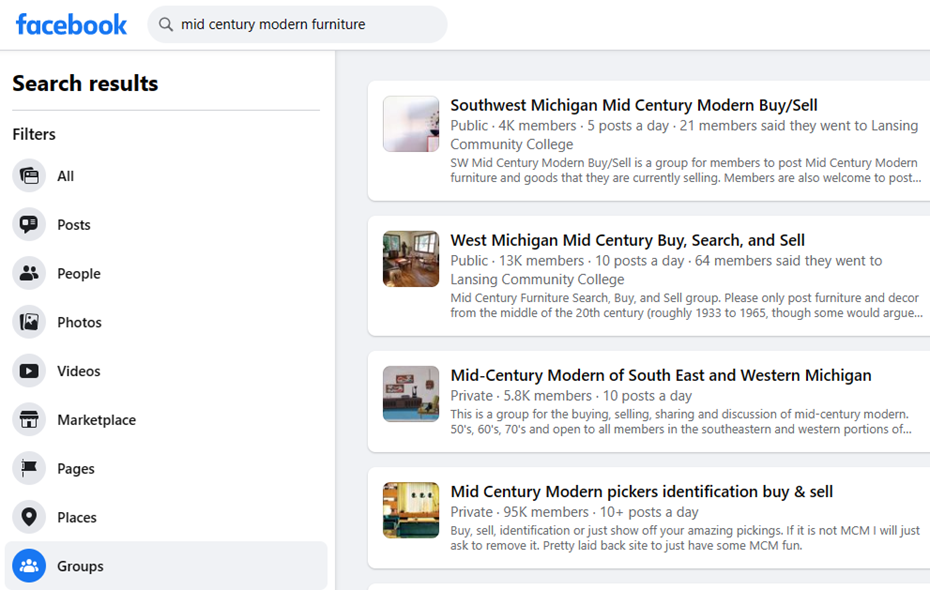The Facebook search results page is displayed on a white to light gray gradient background. Prominently at the top, the iconic "Facebook" logo is presented in its stylized lettering. Adjacent to this logo, on the right, is a gray search bar with a darker gray magnifying glass icon inside, accompanied by the text "Mid-Century Modern Furniture."

Directly below the search bar is a vertically oriented menu bar. The first item, "Search Results," is prominently displayed in black, followed by "Filters." Below these, a series of options are listed with corresponding icons to the left: All Posts, People, Photos, Videos, Marketplace, Pages, Places, and Groups. The "Groups" option is highlighted in blue, distinguishing it from the rest, which are in gray.

On the right side of the menu, the search results focus on Facebook groups related to Mid-Century Modern furniture in various regions. The highlighted group, "Southwest Michigan Mid-Century Modern Buy/Sell," is followed by other similar groups: "West Michigan Mid-Century Buy, Search, and Sell," "Mid-Century Modern of Southeast and Western Michigan," and "Mid-Century Modern Pickers Identification Buy and Sell." Each group listing includes details such as whether the group is public or private, the number of members, daily post frequency, and a brief description. To the left of each group listing, small profile picture icons are displayed.